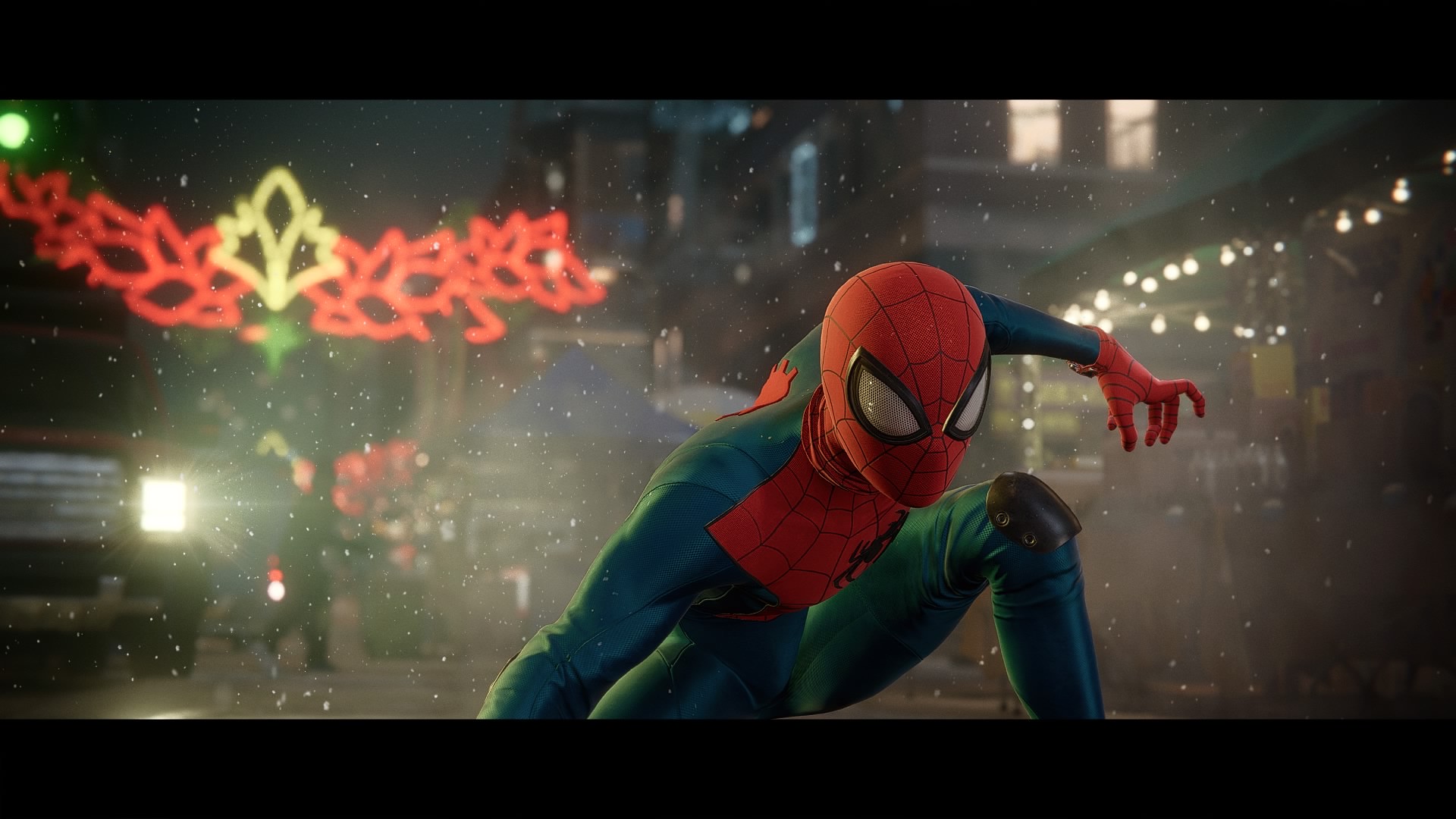The image depicts Spider-Man in his iconic blue and red suit, reminiscent of Tobey Maguire's portrayal of the superhero. Spider-Man is captured in his classic pose: crouching low to the ground with one knee bent and the other knee up, one arm balanced on the ground, and the other poised in the air, exuding a menacing and ready-for-action aura. It appears that he has just landed after swinging through the city, as suggested by his dynamic posture and the wet, rainy atmosphere around him.

The backdrop reveals a dark, possibly nighttime setting with rain pouring down, adding a dramatic effect to the scene. A car is visible behind Spider-Man, indicating that he is either on or near a road. To his left, several buildings can be seen, their details somewhat obscured by the rain. Notably, there is a festive decoration in the background, featuring red and gold lighting, hinting that it might be around Christmas time.

Though the exact scene or movie from which this image originates is unclear, it could potentially be from a movie or an AI-generated creation. Regardless, the atmospheric details and Spider-Man's striking pose make for an evocative and eye-catching image.